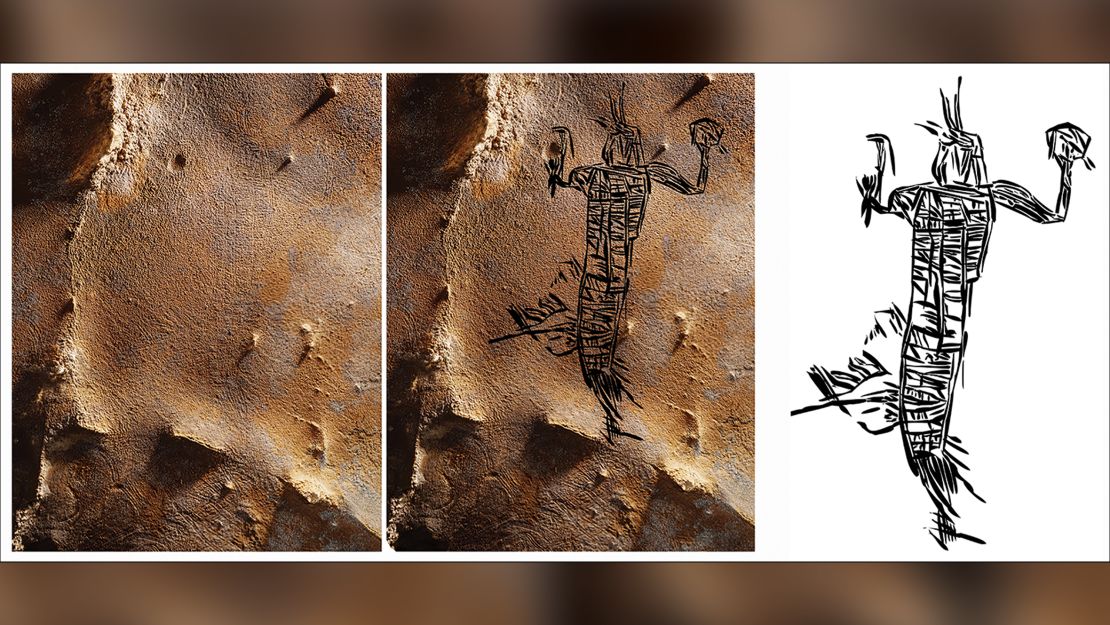The image is composed of three panels that depict the progressive stages of a drawing. The first panel features an earthen wall, possibly a cave or mountainside, with a rough, multi-colored surface that includes holes and ridges. In the second panel, a black, abstract drawing appears on the same wall. The drawing resembles a mix of a scarecrow and a man with indistinct facial features, raised arms, and a body that suggests a single garment enclosing its legs. There are differing interpretations; some see a lizard-like figure, while others describe it as an Indian holding items in both hands. The final panel showcases the completed drawing isolated on a white background, surrounded by a gradient of brown and black. The overall aesthetic suggests a step-by-step reveal of the drawing.